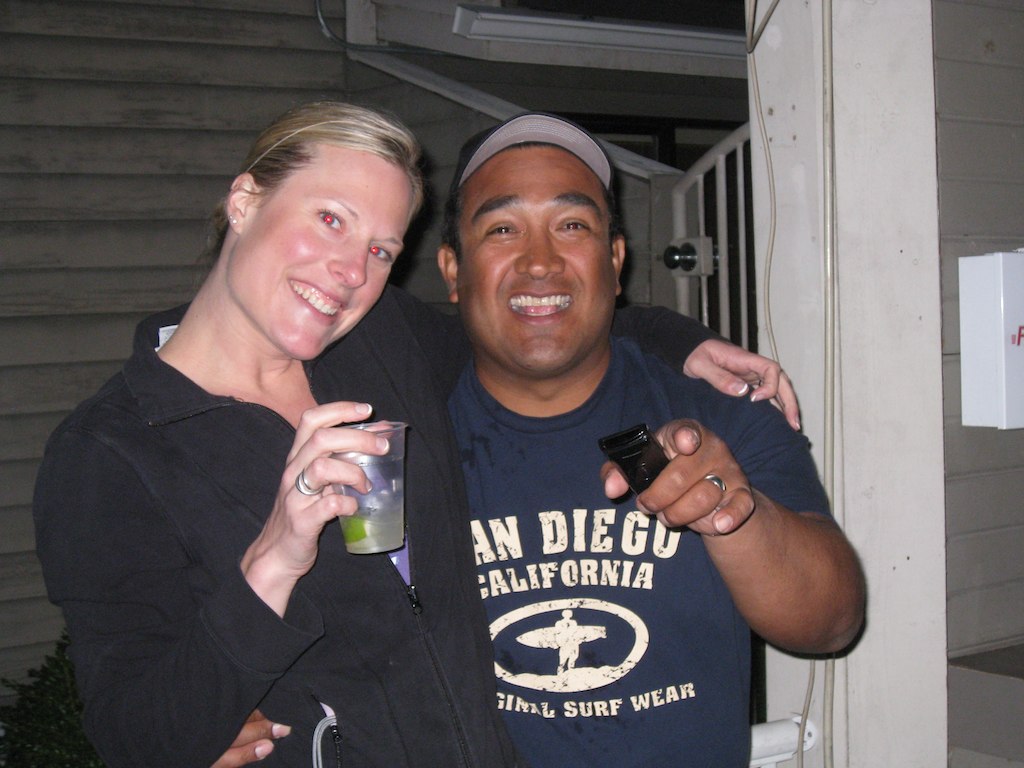In this image, two people are standing together in front of a building, which appears to have wooden horizontal slats, possibly on a porch. The scene is centered around a pair posing closely, right in front of what looks like a gate leading to the outside. The man, who is situated in the center of the frame, is wearing a blue t-shirt with white text that reads "San Diego, California" and features an oval surfer logo followed by “Original Surfwear.” He has a baseball hat on and is smiling warmly at the camera. His right arm is wrapped around the waist of the woman standing to his left, while his left hand points toward the camera, holding what seems to be a television remote or possibly a cell phone.

The woman, standing to the left of the man, is grinning widely, showing all her top teeth. Red-eye from the camera effect is noticeable in her eyes. She has her hair pulled back and is dressed in a black collared jacket. In her right hand, she’s holding a clear plastic cup containing a clear liquid with a lime floating in it. She's also wearing a ring on her right ring finger. Her left hand rests over the man’s shoulder, completing their close pose. There is a white post visible above the man's left shoulder, and a white box, potentially an emergency box, is attached to the wall to their right. Additionally, something that looks like a cord or string is peeking out from the pocket of the woman's jacket.